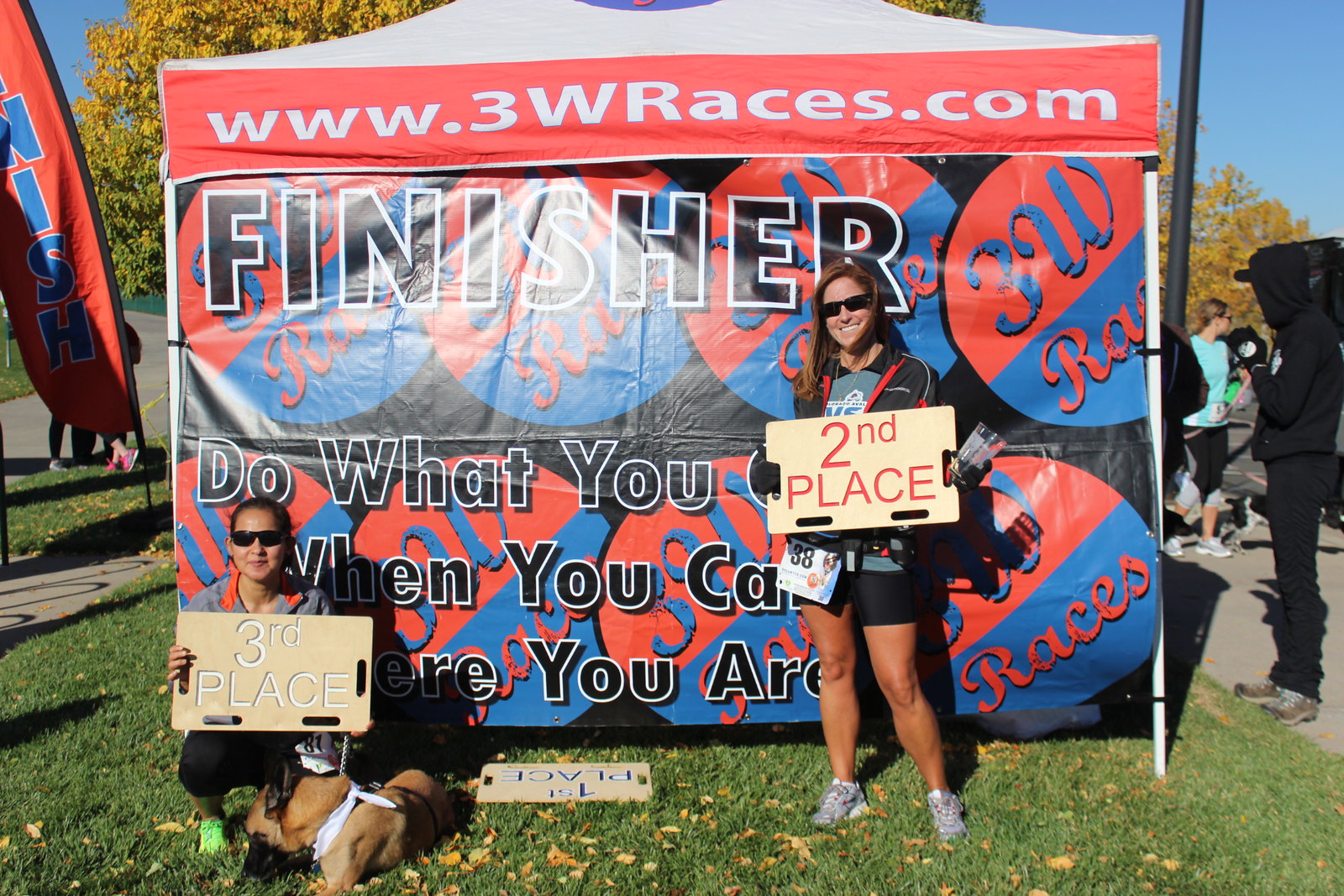In this vibrant outdoor photograph, two women and a German Shepherd are positioned in front of a pop-up tent adorned with a prominently displayed banner. The banner features the website URL "www.3wraces.com" in white letters against a red background at the top. Below it, the words "finisher do what you" are visible, partially obscured by the women.

The woman on the left, who has black hair, black glasses, a gray shirt, and black pants, is squatting down and holding a "third place" sign. Beside her, lying on the grass, is a German Shepherd. An unattended "first place" sign lies on the ground next to them. The woman on the right, who has brown hair, black glasses, a black jacket, a gray shirt, black shorts, and gray shoes, is standing and holding a "second place" sign.

The backdrop includes a roadway, some trees, a bit of sidewalk on the left, and a gathering of people milling about on a paved area to the right. Additional banners and the serene environment contribute to the celebratory atmosphere of the scene.